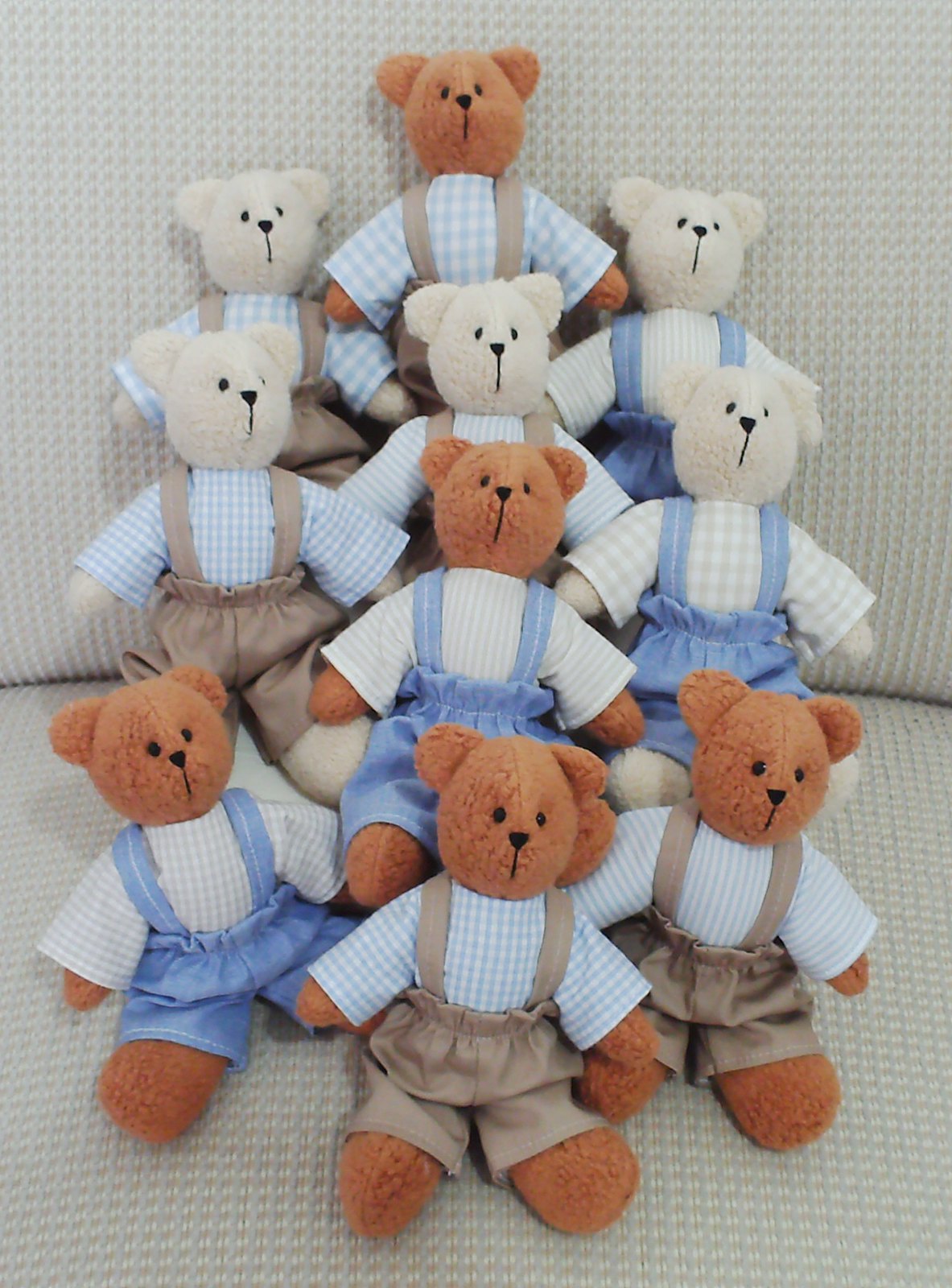This close-up photograph showcases a charming collection of ten teddy bears, meticulously arranged on a white, fabric-textured couch adorned with a small blue and light brown embroidered design. The teddy bears are divided equally by color, featuring five with chocolate brown fur and five with white fur. They are all dressed in overall shorts coupled with long-sleeved, button-up shirts in varying plaid patterns.

Each teddy bear's face is characterized by black, circular eyes, a small upside-down triangle for a nose, and a simple seam that forms a line descending from the nose to signify the mouth. The overalls differ in color; some are khaki brown while others are denim blue. The chocolate brown teddy bears wearing blue suspenders don lighter plaid shirts—one with plaid lines and another with a striped pattern. In contrast, those in tan suspenders exhibit cyan blue shirts, also varied in plaid and stripe designs.

Similarly, the white teddy bears with tan suspenders feature plaid shirts, some with broader spacing of blue plaid stripes and others with regular blue and white stripes. Those in blue suspenders don beige-striped and beige-plaid shirts. The arrangement on the couch is deliberate, with groups and rows highlighting the mix of colors and outfits. In the front, two chocolate brown teddy bears with blue suspenders sit before a group of three white teddy bears. Overall, this delightful scene captures the harmonious diversity in appearance yet uniformity in style among the teddy bears.